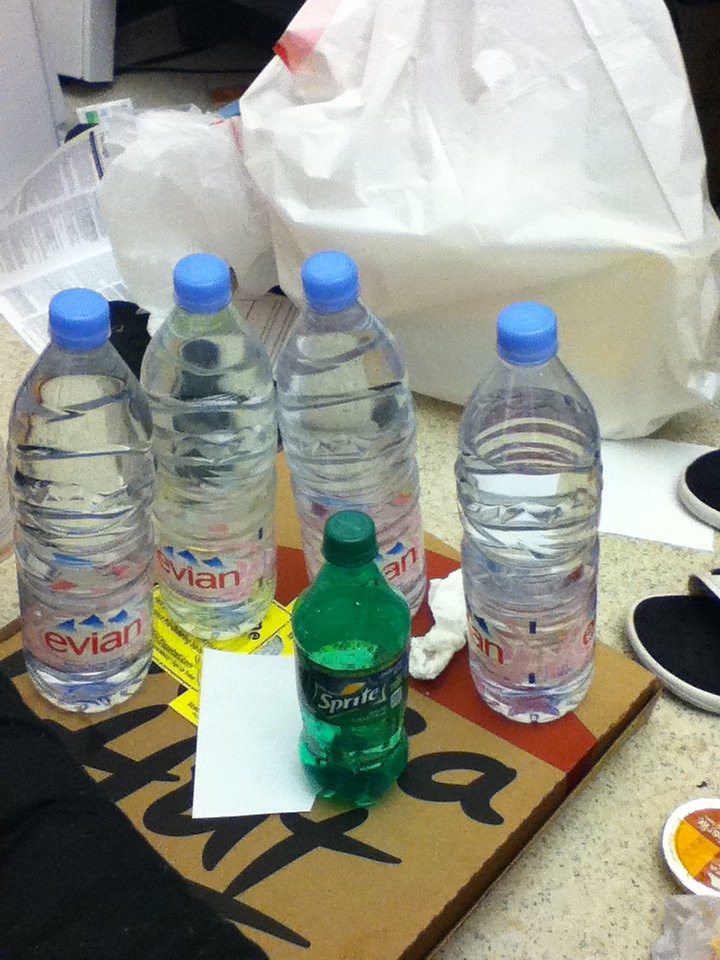This detailed photograph depicts a cluttered kitchen countertop featuring a partially consumed Pizza Hut meal amidst various items. Dominating the scene is a manila-colored Pizza Hut box, marked prominently with the iconic red roof logo. Scattered atop the box are a crumpled napkin, an upside-down receipt, and some unidentified yellow and white papers. Arranged around the pizza box are four tall Evian water bottles, three of which are full, while one appears to have been partially consumed. The bottles have their characteristic electric blue caps and white labels emblazoned with red ‘Evian’ text. Near the center of the box sits a small, mostly empty green Sprite bottle with a green cap and a yellow-green citrus label.

To the right of the composition, there is a small, unopened dipping sauce container with a silver foil top revealing a yellow interior. Additionally, there is evidence of two items of footwear—a pair of black slides with white soles—positioned near several plastic takeout bags. The bags are filled with papers and other miscellaneous items, contributing to the overall sense of disarray. The surface on which everything is placed is a kitchen countertop, yellowish-white with black speckles, which contrasts with the random clutter of objects littering the space.